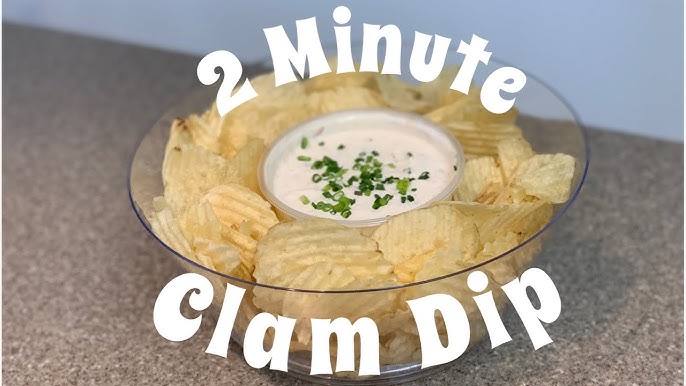This photograph captures a transparent glass bowl brimming with yellowish ruffled potato chips, positioned on what appears to be a burgundy or brown surface, likely a table. Nestled in the center of the chips is a smaller bowl of clam dip, adorned with a generous sprinkle of green onions. Prominent white text is displayed both above and below the bowl, reading "Two Minute Clam Dip." The setting seems to be indoors, and the overall presentation of the dip and chips looks very appetizing.